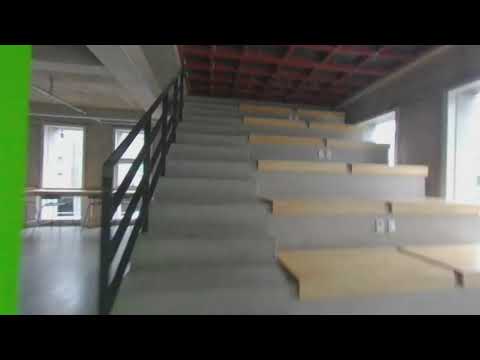The image showcases a vertical rectangular photograph with horizontal black stripes framing the top and bottom. Dominating the picture is a staircase towards the right of the center, ascending upwards. The staircase is predominantly made of gray concrete with light brown wooden covers on each step. On the left side of the staircase, there is a sturdy dark gray metal railing. To the far right of the staircase, the gray wall features several windows.

Adjacent to the staircase on the left side of the image, a long table and several chairs are discernible, though their colors are indistinct. Above, the ceiling is marked by a distinct red and black checkered pattern. Additional elements include what seems to be a grain post on the left edge of the photo and a structure resembling a door next to the black railing. The setting appears to be indoors, perhaps within a school or institutional building, as suggested by the layout and furnishings.